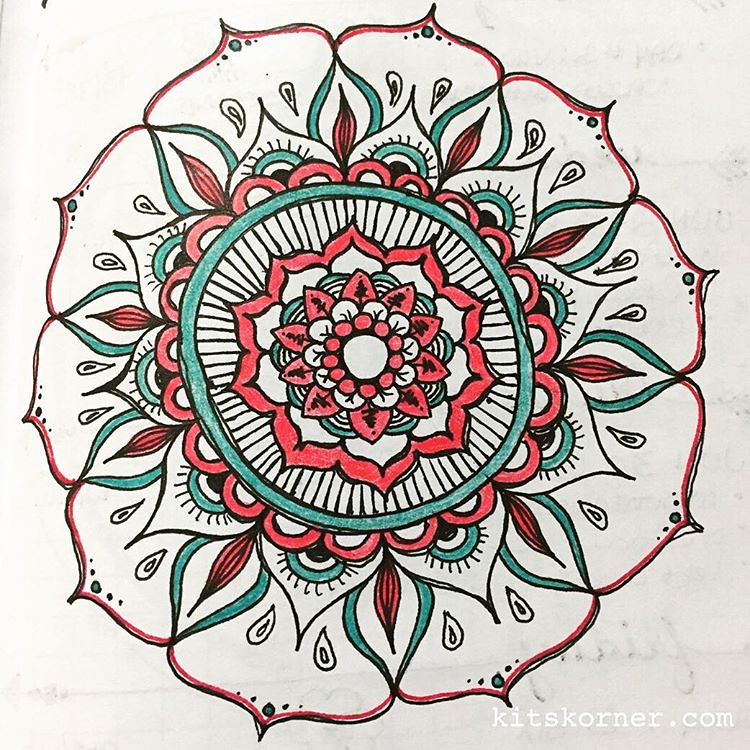This intricately detailed drawing features a floral design set against a white sheet of paper. In the bottom right-hand corner, the website "kidscorner.com" (spelled K-I-D-S-K-O-R-N-E-R dot com) is inscribed. The central bloom is illustrated in hues of red and green, with each layer of petals contributing to its complex structure. 

Beginning with the outermost layer, the red petals are outlined but not filled in. Each of these larger petals contains a green circle at its center. Extending from these circles are two teardrop shapes, leading to another series of slimmer red petals and followed by green petal shapes resembling eyes. Further in are half-circle red petals. At the flower's heart lies a large green circle embellished with lines and containing an additional smaller flower within it, adding further depth and intricacy to this vibrant floral composition.